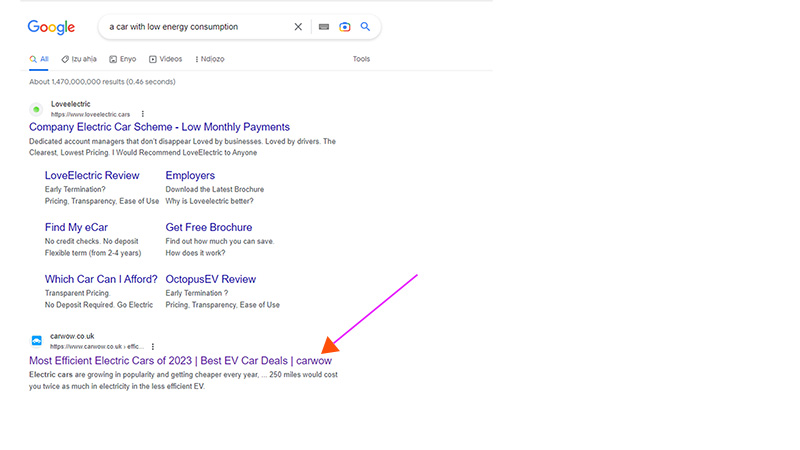The image depicts a Google search results page. At the top, the Google logo is prominently displayed. Within the search bar, the query "car with low energy consumption" is entered. Directly beneath the search bar are the typical filter options: 'All', 'Images', 'Videos', 'News', and 'Tools'. The search yields over 1.4 million results.

The first highlighted search result is for "Love Electric". It describes a company offering an electric car scheme with low monthly payments. This listing includes several links beneath it, such as a detailed Love Electric review, an option to find a car, a tool to determine which car one can afford, information for employers, a link to request a free brochure, and a review of Octopus EV—all related to the Love Electric website.

The second listing, though slightly blurred and difficult to read, appears to be from another UK-based car website. It offers information on the most efficient electric cars of 2023 and the best EV car deals, specifically mentioning "Carwow". There is a red arrow pointing to this entry, indicating it's likely a review site offering extensive product reviews for various electric vehicles (EVs).